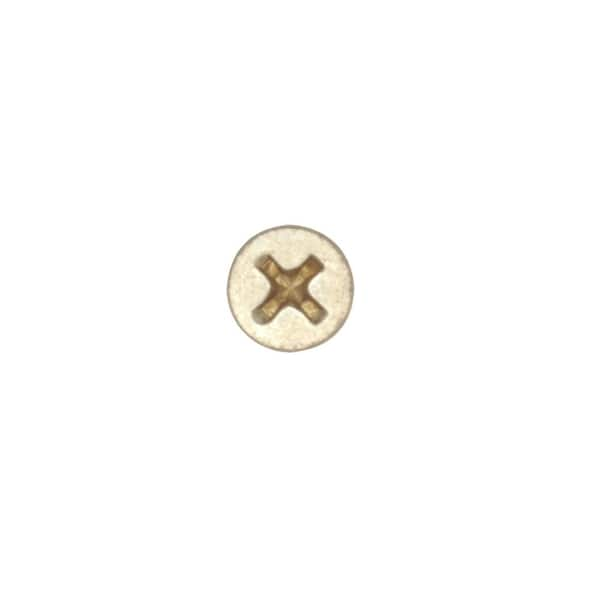The image depicts a minimalistic composition set against a solid white background. At the center lies a circular element bordered by a gray ring. The interior of the circle features a light beige texture, scattered with subtle off-white speckles, adding a slight visual depth. Intricately placed within this circle is a prominent X-shaped design. The X is crafted with wooden aesthetics, showcasing a nuanced color palette: the arms of the X are brown with lighter brown edges, converging at a central point where a blend of white and light brown highlights accentuate the intersection. This simple yet detailed representation could evoke the appearance of a functional button or a screw head, inviting various interpretations. Overall, the image focuses on the central circular motif with its distinct, layered X, framed by the seamless white backdrop.